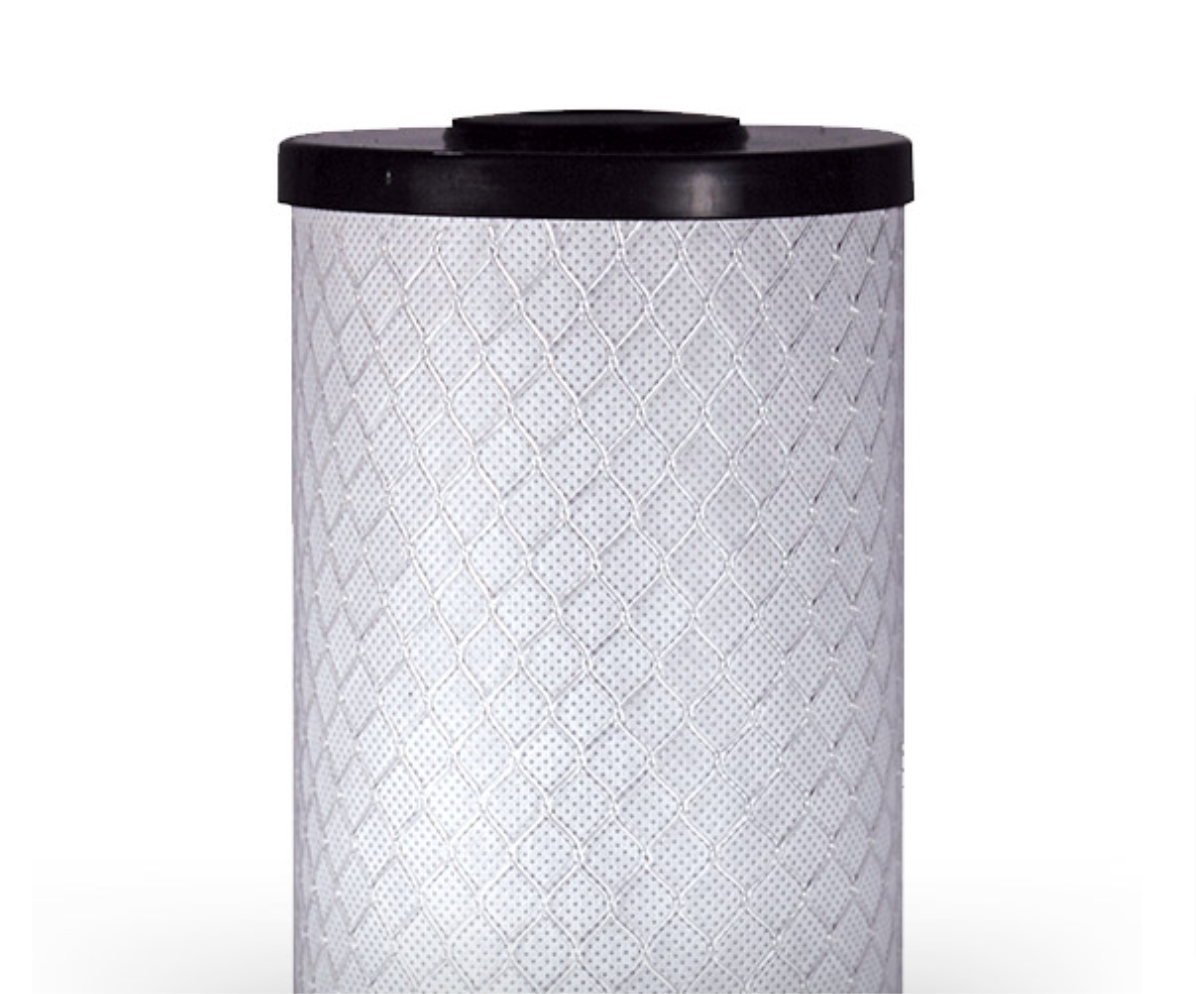This is a close-up photograph of a cylindrical filter standing against a white background. The image captures only the top portion of the filter, with the bottom part cut off. The prominent black plastic cap at the top features a small protrusion. Enclosing the body of the filter is a crisscross mesh of silver metal that forms a diamond pattern. The surface of the filter itself looks like matte white fabric and is covered with uniformly tiny air holes, giving it a detailed and textured appearance. The light shadow on the top of the black plastic cap adds depth to this product-focused image, reminiscent of the detailed views typically seen in online product listings.